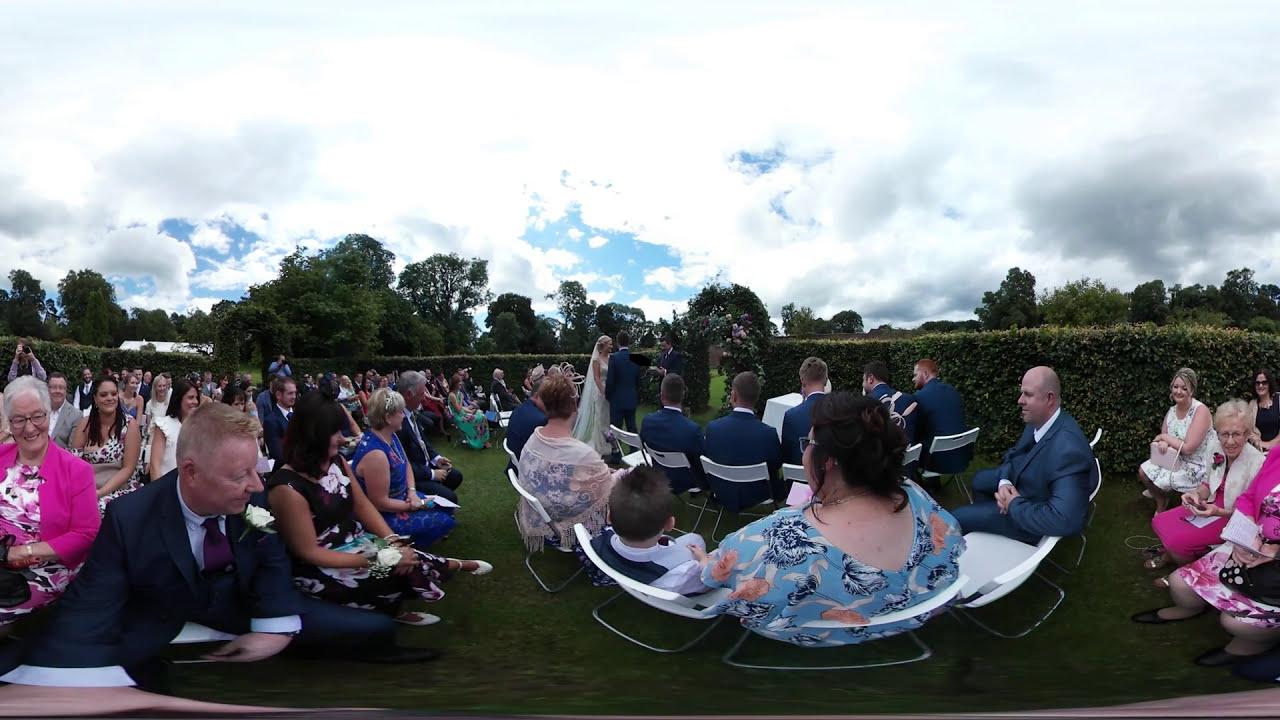The image captures a vibrant outdoor wedding in a lush, green setting. The focal point is the bride and groom standing before a pastor under a beautifully adorned flower archway. The ceremony unfolds against a backdrop of a tall, green hedge, with trees and a building visible in the background, adding to the picturesque environment. The sky is a clear blue with a few clouds, suggesting a perfect summer or fall day. Surrounding the couple are well-dressed guests of all ages, with some elegantly dressed in suits, dresses, and colorful attire ranging from blues and pinks to purples, reds, blacks, and whites. The guests, seated in neat rows of folding chairs, look on with smiles, a few shedding tears of joy. Among them, a notably large woman in a blue dress sits prominently with a child beside her. The setting radiates happiness and celebration, as friends and family gather to witness the couple exchange their vows, encapsulating a joyous moment in a beautifully natural setting.